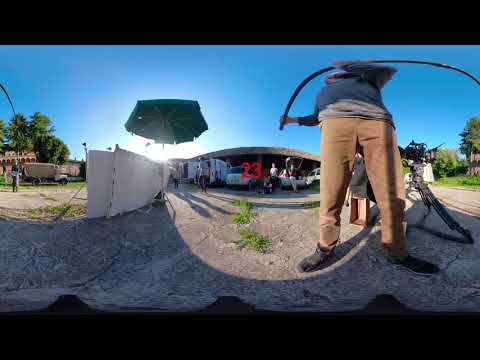In this outdoor photograph, the lower half of a person's body is prominently displayed on the right side, creating a focal point for the image. The individual is dressed in brown khaki pants, a blue long-sleeve sweater over a gray shirt, and brown boots. They appear to be holding a black hose or tube, which looks slightly curved due to the camera's distortion.

The setting is somewhat ambiguous but hints at an open, somewhat public space with a mix of elements. A large canopy umbrella, possibly green, stands to the left against a white wall, and there’s a fence nearby. The background features a brilliant turquoise sky, trees, a brownish building, parked cars, and people walking around. Additionally, there's a roof with the numbers "23" prominently displayed in red, serif font, seemingly superimposed over the image. The ground appears to be cement, and a short plant, roughly knee-height, can be seen near the person's feet.

Overall, the image conveys a vivid, slightly distorted scene with multiple layers of activity and architecture, united by the striking "23" in the center.